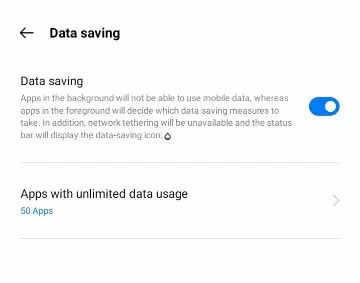This image is a screenshot of a tablet or smartphone screen, focusing on data-saving features. 

On the left-hand side, there's a bold black arrow pointing right. To its right, bold black text reads "Data Saving," with finer black text below repeating "Data Saving." Beneath this, a gray text description explains, "Apps in the background will not be able to use mobile data, whereas apps in the foreground will decide which data-saving measures to take. In addition, network tethering will be unavailable, and the status bar will display the data-saving icon." This icon is depicted as a black teardrop symbol. 

On the right-hand side, a toggle button is shown, turned on, represented by a blue background with a white circle shifted to the right. 

Following this section, bold black text states "Apps with unlimited data usage," accompanied by a right-facing gray arrow. Below this heading, 50 apps are indicated in hyperlink blue text. Each section is separated by a thin gray line. 

The image lacks any visible scroll bars, navigation buttons, or top menus, except for a back arrow, suggesting the top, bottom, left, and right edges are cut off in the screenshot. Given the compact nature of this screenshot, it likely originates from a smartphone.